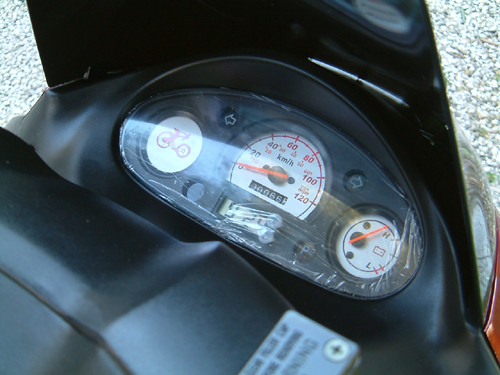The control panel of an electric scooter features a more or less oval design, anchored by three prominent circular gauges. The central gauge houses an LCD display beneath it, though the exact text on the display is not discernible. Above this LCD is a speedometer with a red needle, calibrated in both kilometers and miles per hour. Flanking the speedometer are circular turn signal indicators. On the left-hand side of the panel, there is another circular LCD screen displaying an image of the scooter, which might be customizable. To the right, there is a gauge with a battery symbol, marked with the letters "H" and "L" for high and low, and it features a red needle indicating the battery level.